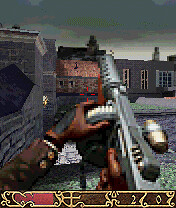The screenshot from a first-person shooter game captures an outdoor urban scene with an overcast, gray sky, evoking a desolate atmosphere. The player's perspective shows only the forearms and hands of the character, who has dark skin and is clad in long leather sleeves and brown gloves. The hands grip a Thompson machine gun with an ammo drum, aimed with a small red crosshair in the center of the screen. The background consists of European-style buildings, predominantly gray stone structures. To the left, there is a large red brick house, followed by another building made of cinder block. One of the buildings features several large windows and a chimney. In the foreground, a small patch of grass peeks through the scene. The bottom of the screen displays a user interface with gold-trimmed menu areas, a health bar denoted by a long red section, and additional indicators with numerical values. The overall composition emphasizes a bleak, war-torn environment typical of many conflict-themed video games.